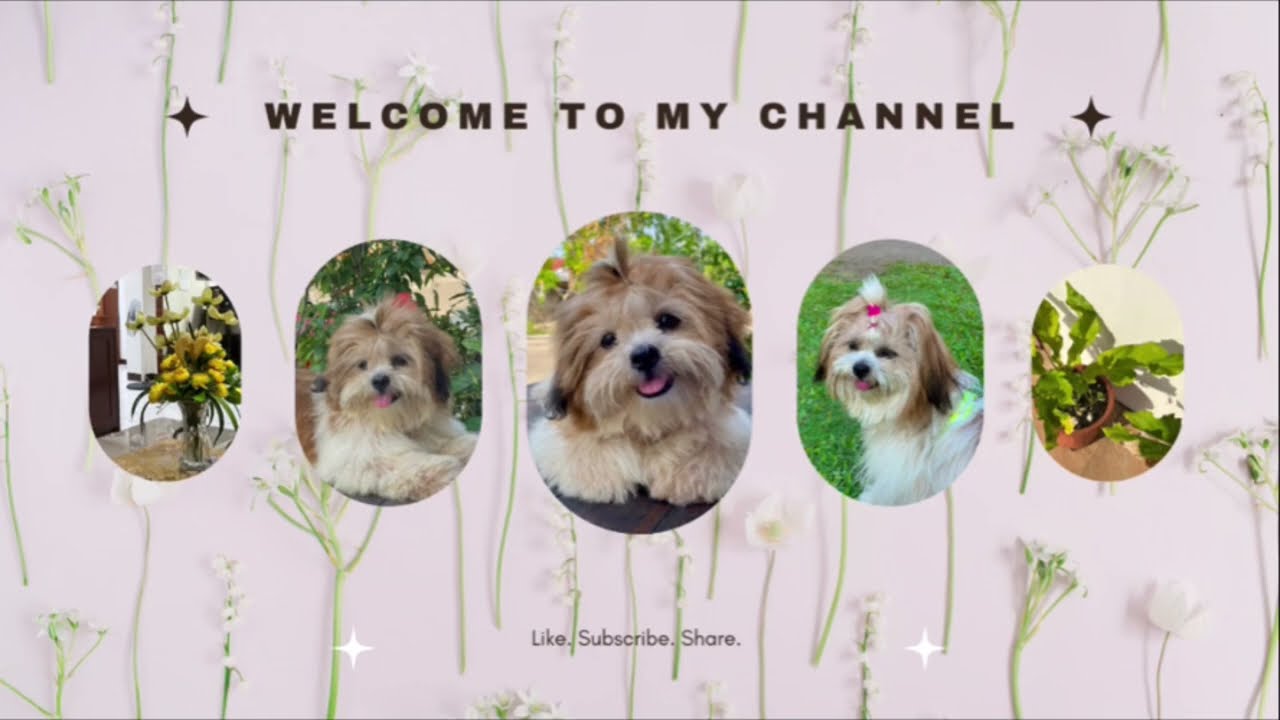The image is a welcome or splash screen for a website or video channel with a cute and inviting aesthetic. The background features hand-drawn trees and plant life with various flowers, creating a natural and cozy setting. In the center of the horizontal rectangular image, there are five oval panels arranged in a row, smaller at the ends and gradually larger towards the middle. 

The first oval on the left is small and contains a bright sunflower against a neutral backdrop. Next to it, the second oval is slightly larger and shows an adorable Lhasa Apso dog with a white body and muzzle, brown patches over its eyes and ears, smiling with its tongue sticking out. The central and largest oval displays the same Lhasa Apso, this time with its head tilted to the left, smiling, and showcasing its charming white paws under its chin. The fourth oval, which is the same size as the second, features the dog in a grassy field with a bow or ponytail on top of its head, looking towards the camera at a three-quarter angle. Lastly, the fifth oval on the far right, the same size as the first, shows a green leafy plant.

Above the ovals, centered horizontally, is the black text "Welcome to My Channel," adorned with diamonds on either side. Below the ovals, also centered, is smaller black text that reads, "Like, Subscribe, Share."

The colors in the image include white, brown, tan, red, green, beige, yellow, pink, dark gray, and black, complementing the natural theme with visually appealing contrast and warmth.